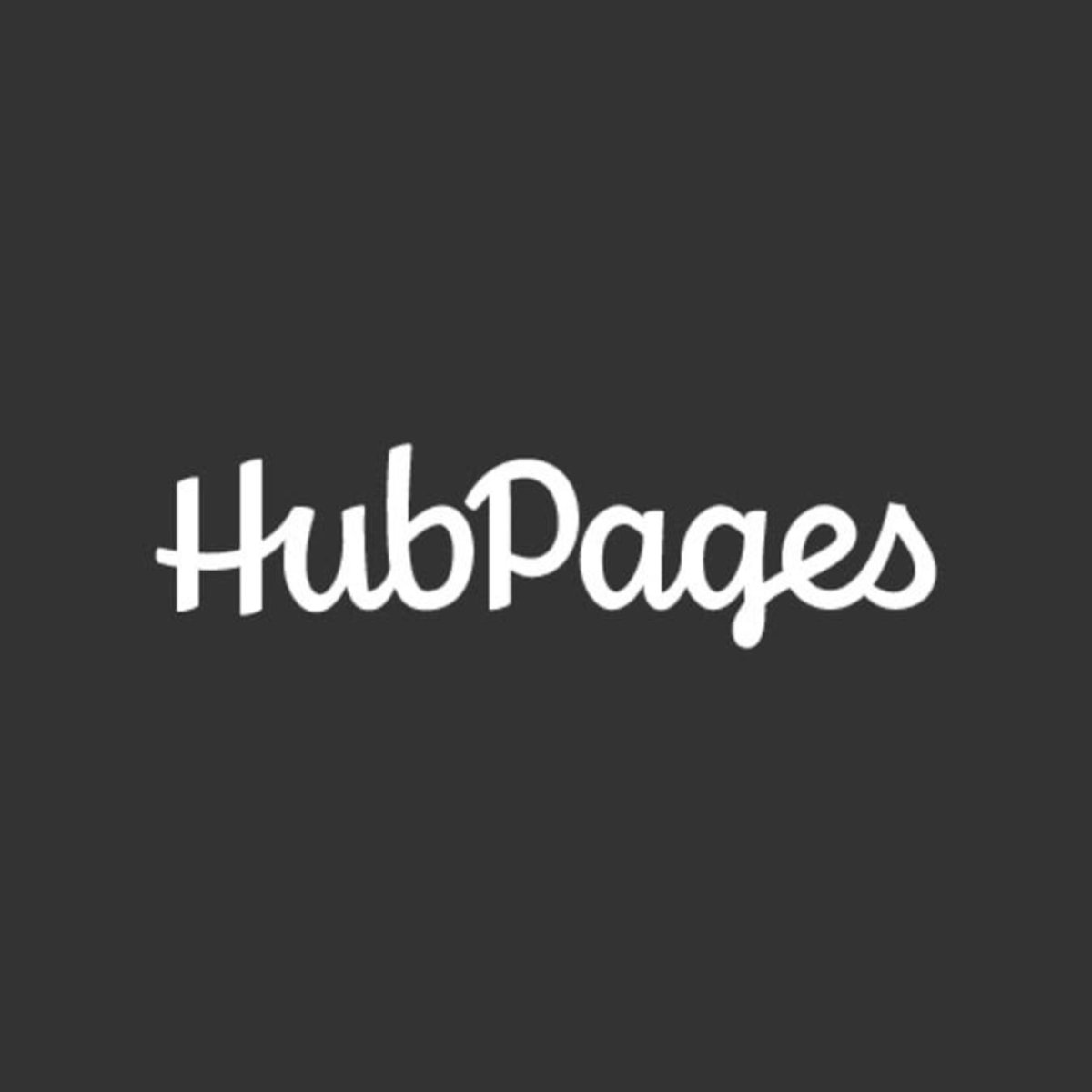The image is a minimalist graphic featuring a solid black square background. Positioned centrally in the square is the word "HubPages," displayed in a white cursive font. The text "HubPages" is capitalized, with both the "H" in "Hub" and the "P" in "Pages" distinctly prominent. There are no additional elements such as images of people, animals, plants, buildings, flags, signs, vehicles, or any other objects. The design is strictly limited to the black background and the white cursive text, providing a clean and simple aesthetic.